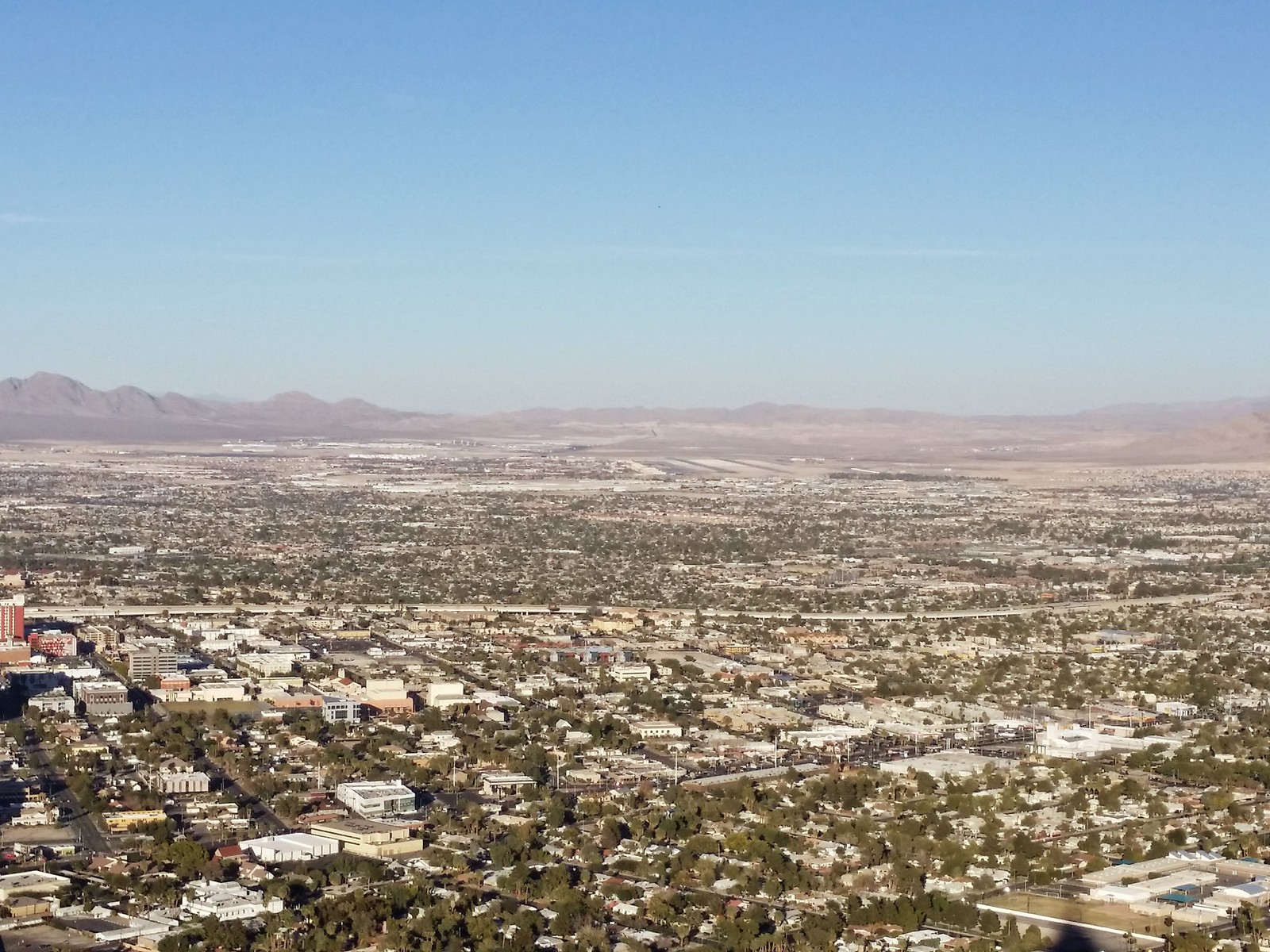A breathtaking wide-angle aerial shot taken from either a drone or a helicopter captures the vast expanse of a bustling city. The image offers a comprehensive view encompassing diverse areas including suburban neighborhoods, bustling business districts, and intricate city streets. A major highway runs prominently through the heart of the urban landscape. The scene is dense with thousands of buildings, each contributing to the complex mosaic of this sprawling metropolis. 

In the far background, the cityscape gradually gives way to arid, desert terrain. The sandy dunes and stark, treeless hills convey the harsh beauty of the desert, with the silhouette of small, rugged mountains dotting the horizon. Dominating the distant center of the image is a large runway, indicating the presence of a significant airport, further underscoring the city's role as a vital hub of activity.